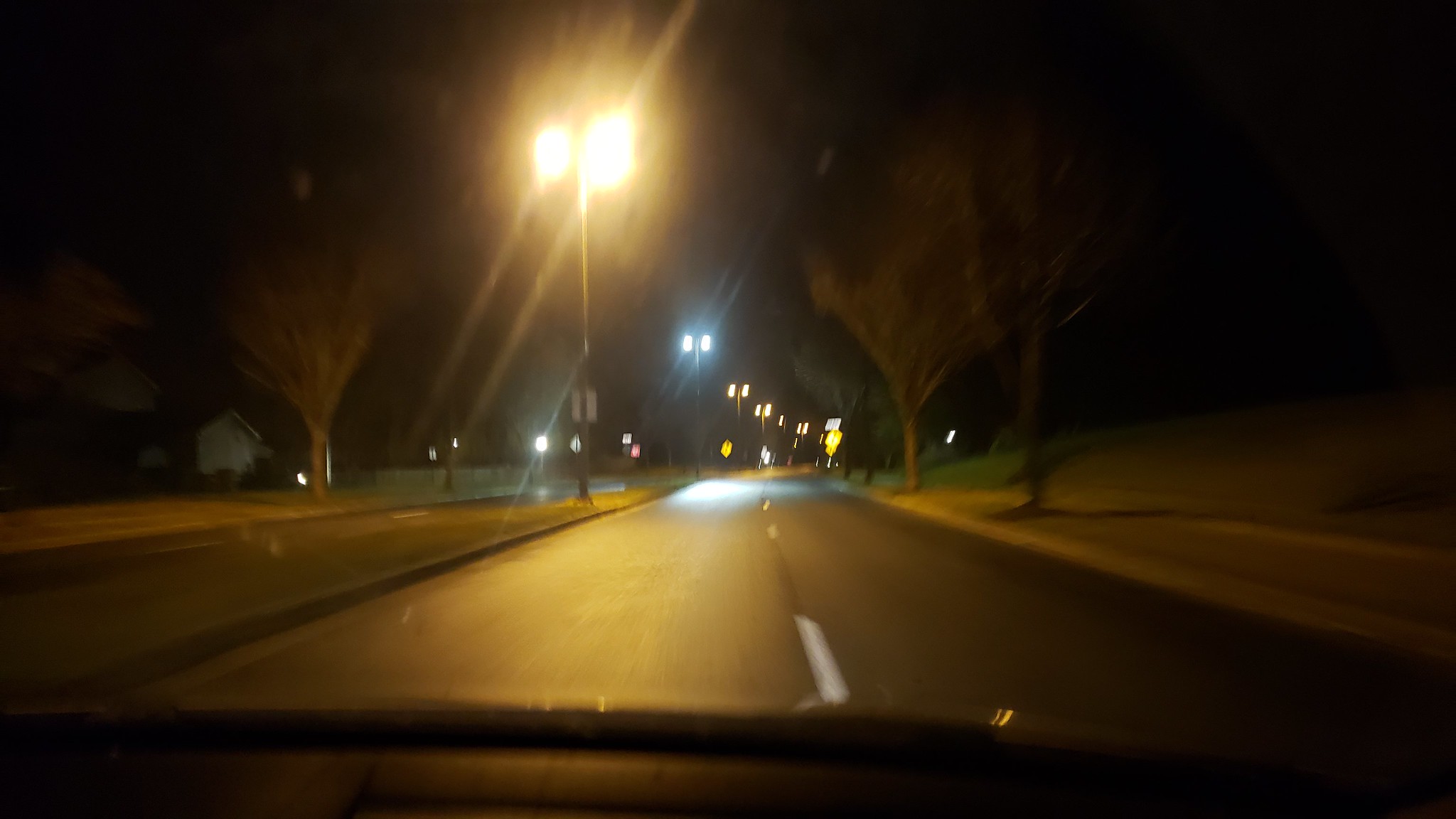A blurry dashcam image captures a nighttime scene from a car driving at speed. The streetlights emit a soft, halo-like glow reminiscent of the visual distortions experienced by those with astigmatism. The road markings are streaked, indicating the vehicle's motion. In the blurry distance, a few houses are barely discernible in the darkness, offering no illumination. The road ahead is clear, devoid of oncoming traffic, and the car's interior remains shrouded in darkness.